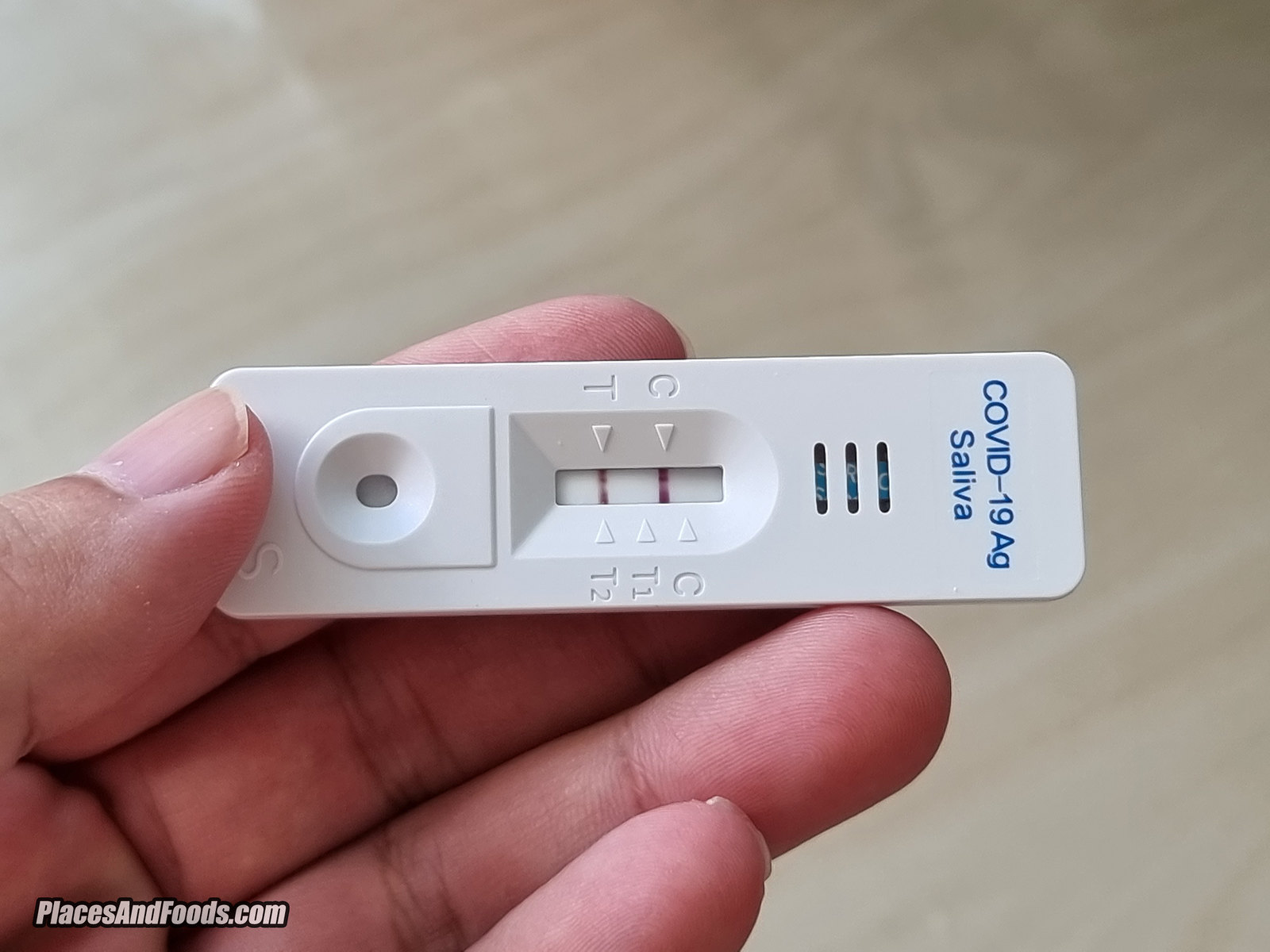In the image, a hand delicately holds a white plastic COVID-19 test over a light birch wood table. The test is a long, rectangular device with rounded edges, approximately a quarter of an inch thick. The text "placesandfoods.com" is visible in the bottom left corner of the photograph. The test is marked with "COVID-19 AG Saliva" written in blue ink at the top, prominently indicating its purpose. 

Three designed slits are present on the device, part of the test’s mechanism. These slits encompass a deep well, labeled with a ‘C’ (for control) and a ‘T’ (for test). In this particular case, there are two red lines, indicating a positive result for COVID-19. Further down the device, an oval-shaped well marked with an 'S' is where the saliva sample would have been deposited for testing. The image captures the details and intricacies of the test, with the hand’s positioning providing a sense of scale against the backdrop of the wooden table.